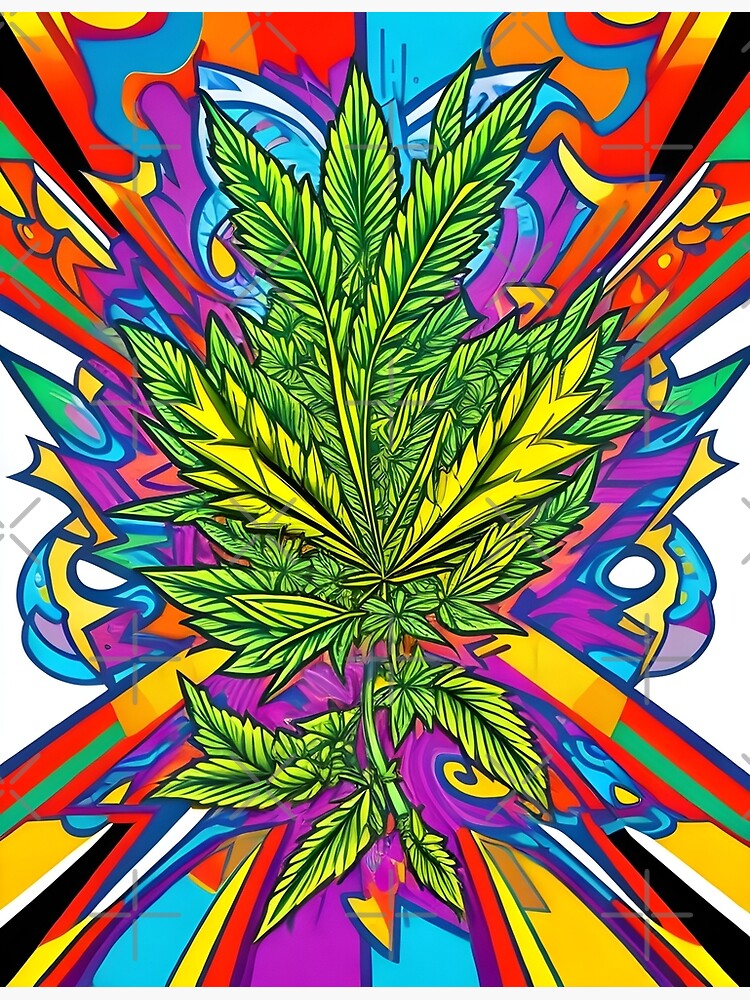The image is a vibrant, psychedelic poster featuring a striking composition of marijuana leaves at its center. The middle of the poster showcases multiple marijuana leaves layered over one another, with the foremost leaf depicted in a light lime green with hints of yellow, while the leaves behind are darker shades of green. Surrounding these central leaves is an explosion of vivid, abstract colors radiating outward in a star-like pattern. The colors streaming from the center to the outer edges include bright reds, greens, purples, yellows, oranges, blues, pinks, and whites, creating a kaleidoscopic effect. The colors burst out at varied angles around the top and bottom, but more mixed and subdued toward the left and right sides. The entire display is set against a white border, heightening the poster's dynamic and animated cartoon-like quality.